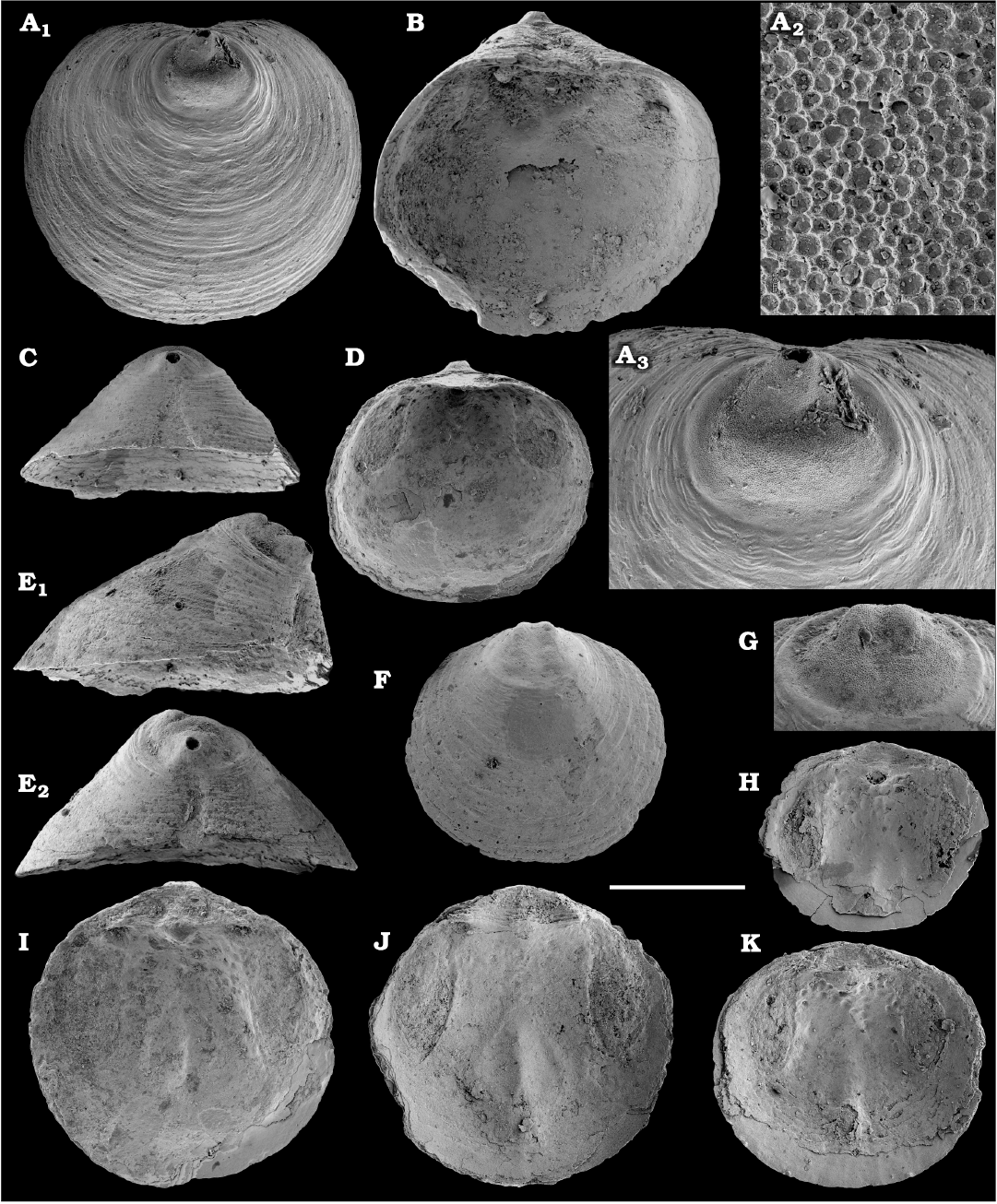This image is a grayscale collage depicting multiple views and angles of what appear to be seashells or rock formations, displayed against a black background. The layout is segmented and labeled from A1 to K, with each section featuring close-up, high-resolution photographs. 

- In the top left corner, A1 shows a circular object adorned with fine spiral patterns, likely a top-down view.
- To the right, image B reveals what resembles the underside of the object shown in A1, characterized by a crater-like depression.
- A2, positioned at the top right, presents a macro shot displaying numerous small gray dots.
- Below A1, image C offers a side profile of a triangular formation.
- Images labeled E and E2 depict triangular pieces of the objects, contributing to the overall fragmented rock appearance.
- Image D, similar to B, also shows a carve-out, possibly another perspective of the crater-like feature.
- In the bottom row, A3 and the remaining labels F, G, H, I, and K show various textures and patterns—ranging from intricate spirals to dot clusters—which adds to the visual complexity.
- The bottom section contains three prominently circular rocks, with additional triangular and smaller circular forms arranged above them.

The objects throughout the image vary in their visual texture and dimension but maintain a coherent color scheme of gray with hints of white and black. The diverse angles, close-up shots, and repetition suggest these might be different perspectives of the same seashell or rock formations, allowing for detailed examination of their intricate natural patterns.